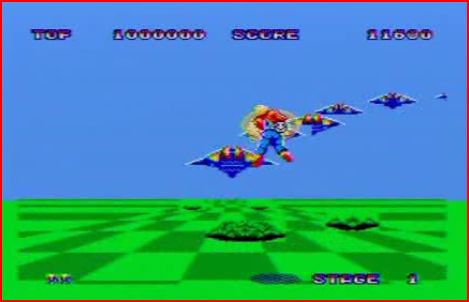This screenshot from a computer or video game features a detailed visual composition. At the top of the screen, there is a line of text displaying "Top 1,000,000" and "Score 11,600" from left to right, indicating the player's ranking and current score. A thin red border frames the entire screenshot, adding a distinct boundary to the image. The scene itself presents a checkered terrain in light green and dark green hues, set against a medium blue sky. A character is seen flying in mid-air, distinguishable by their red shirt, blue pants, and red shoes. Additionally, five small planes are also airborne, dispersed throughout the sky, adding a dynamic element to the setting.